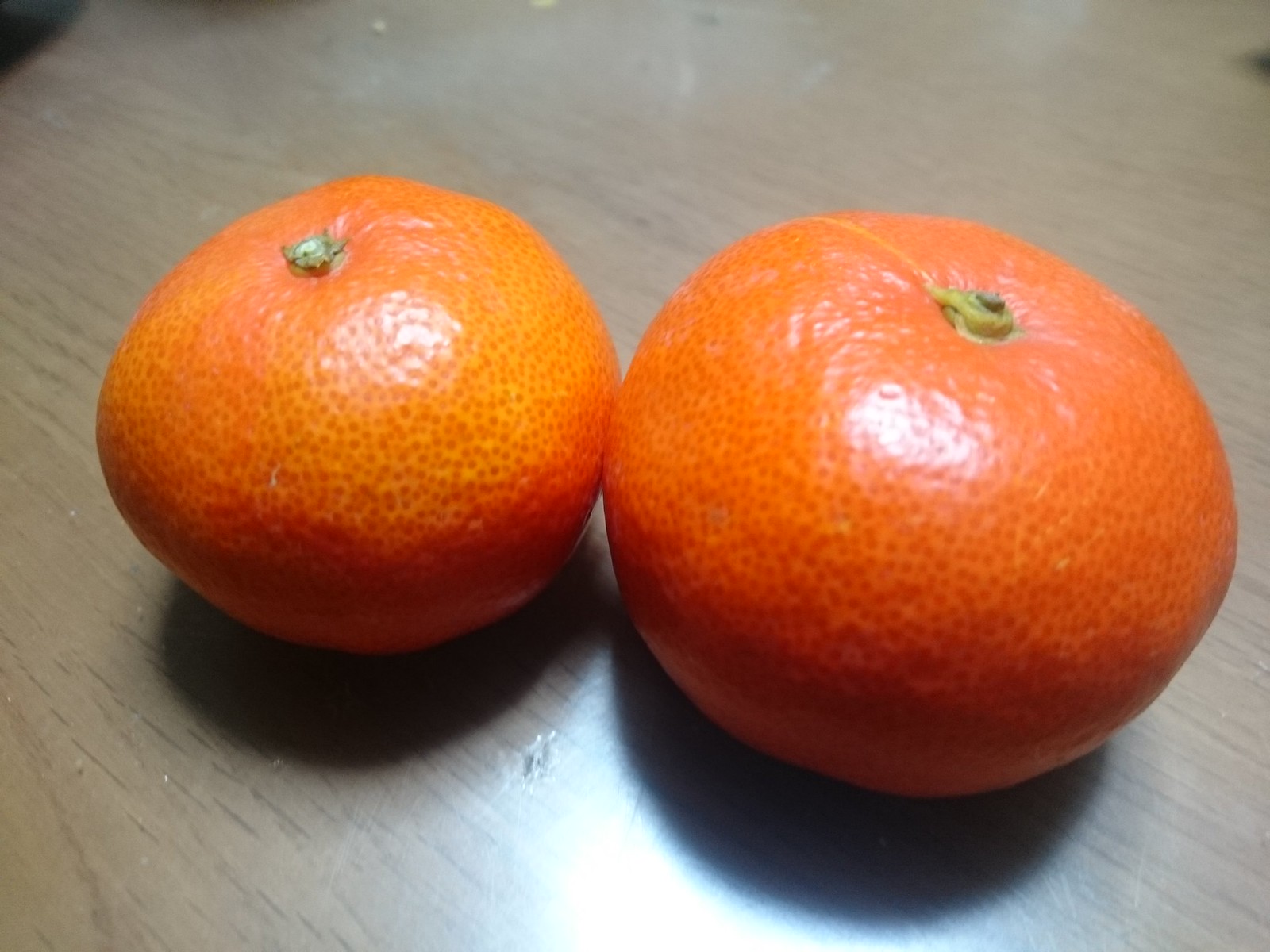This image captures a close-up of two oranges on a light brown wooden countertop that has a faux wood finish. The oranges, set against this tan-brown surface, display varying shades of orange, with the left one being smaller and more traditionally orange, and the right one larger and slightly redder, which suggests they might be blood oranges. Both oranges have light green stems indicating freshness, and their textured skins feature tiny dimples.

Overhead lighting creates reflections and distinct shadows, accentuating the vivid orange hues and revealing a white spot on each fruit where the light hits directly. This lighting also casts deep shadows beneath the oranges and towards the left, emphasizing their round shapes and positioning them as the focal point of the image.

On the countertop, there is a notable small gouge between the fruits, along with some food remnants and minor marks scattered around. Additionally, faint black and green speckles are visible on the wood surface, which suggest a rustic and slightly worn texture. In the image's composition, there are shadows on the upper corners—top left possibly from the table edge and top right from an unidentified object, adding depth to the scene.